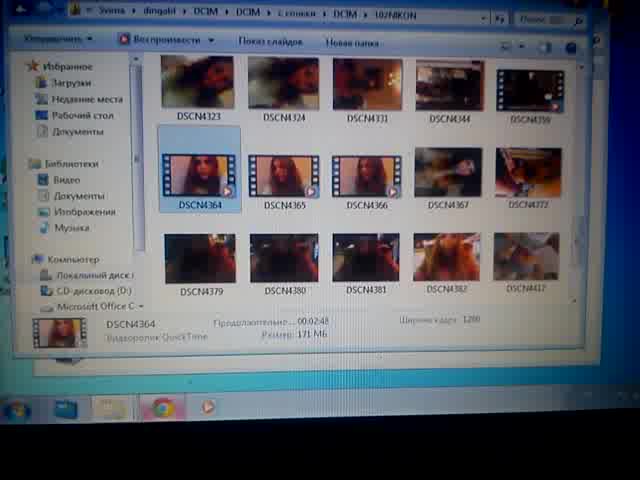The image appears to be a blurry screenshot taken of a computer screen, possibly captured with a digital camera or phone. The screen, displaying the old Windows 7 user interface, features the familiar glossy, blue chrome aesthetic. It shows a Windows Explorer window, specifically a DCIM folder containing several photos and videos. The photos appear to depict a pale woman with brown shoulder-length hair, although the details are indistinguishable due to the pixelation and blurriness. Each file has an auto-generated name starting with "DSCN" followed by a series of numbers, such as DSCN323 and DSCN4364. The UI includes elements in the Russian alphabet, indicating it is in Russian. The bottom section of the screen mentions "Quick Time," also written in Russian. On the left side, there are various black icons with unreadable labels, and the taskbar shows icons for Google Chrome and other possibly Mac-related applications. The top of the screen features a blue border with unreadable text, possibly part of the browser window or another application.